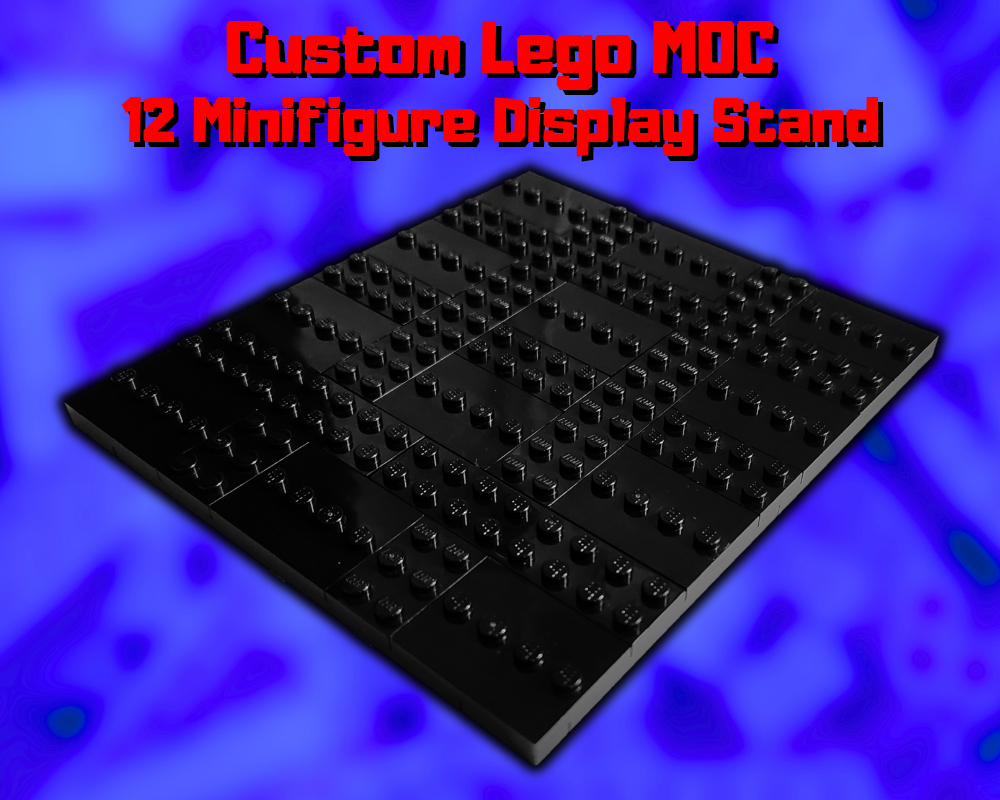The image is a digitally enhanced advertisement for a custom Lego MOC 12 minifigure display stand. The background is a wide vertical rectangle with blurred shades of blue, including dark and light tones, creating a metallic, industrial look. In the center of the image, slightly angled to the right, there is a horizontal flat black plastic stand featuring raised rectangular bumps arranged in a grid pattern, designed for displaying Lego minifigures. This stand appears to be floating due to its placement on the diagonal with the corner facing the bottom left. Above the stand, large bold red text with a black drop shadow reads "Custom Lego MOC 12 Minifigure Display Stand." The image combines photographic realism with representationalism, emphasizing the product's utility and design.